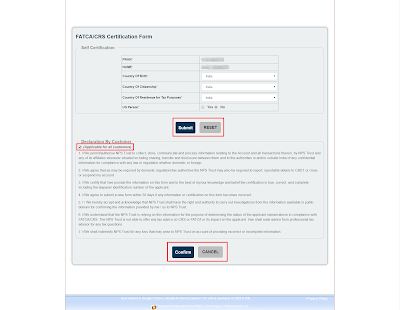The image is a small, blurry, and hard-to-read screenshot of a website, prominently featuring a large square with a light gray background in the center. The overall background of the image is white. At the top of the gray square, in black text, it appears to say "Fat Caucus Certification Form." Below this title, there are several options, dialog boxes, and drop-down menus allowing users to select different settings on the website.

The image highlights specific sections with red outlines, clearly intended to guide users. In the center and lower center of the screen, there are two red-outlined boxes containing buttons. The first red-outlined box, located in the center, includes a blue "Submit" button and a gray "Reset" button. The second red-outlined box at the bottom contains a blue "Confirm" button and a gray "Cancel" button.

Additionally, another section of text or a dialog box on the left-center of the screen is highlighted in red, though its contents are unreadable due to the image quality. The red highlights seem to serve as instructional guides, likely indicating important areas or functions for the user to note while navigating the website.